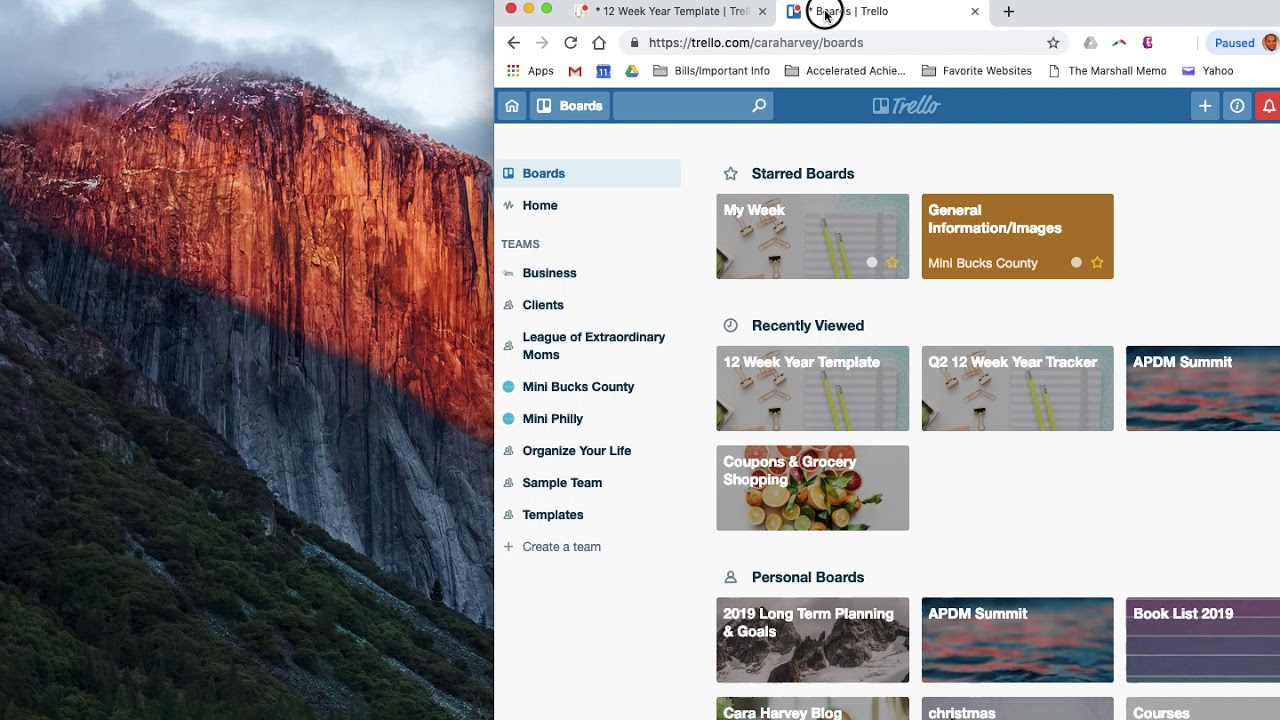The image depicts a website interface set against a background featuring a picturesque mountain range. The mountains are partially snow-capped, with snow concentrated towards the peaks and extending down the sides into shaded areas. The website appears to be Trelio.com, specifically Cara Harvey's set of boards, as indicated by the URL displayed on the screen.

At the top-center of the interface, there is a rectangular area displaying the word "Trelio" in cursive script. The interface highlights various "starred" boards, including "My Week," "General Information / Images," "Mini Bucks County," and the recently accessed "12-week year template," "Quality 2 12-week year tracker," "APDM Summit," and "Coupons and Grocery Shopping."

Scrolling further down reveals the "Personal Boards" section, listing items such as "2019 Long-Term Planning and Goals," "APDM Summit," and "Booklist 2019," although the last entry is partially cut off at the bottom of the image.

Returning to the top of the screen, there is a navigational area with categories labeled "Boards," "Teams," "Business Clients," "League of Extraordinary Moms," "Mini Bucks County," "Mini Philly," "Organize Your Life," "Sample Team," and "Templates." At the bottom of this section, there is an option to "Create a Team."

Overall, the image captures a comprehensive view of the Trelio website interface, showcasing both navigational elements and content organization against a stunning mountain backdrop.